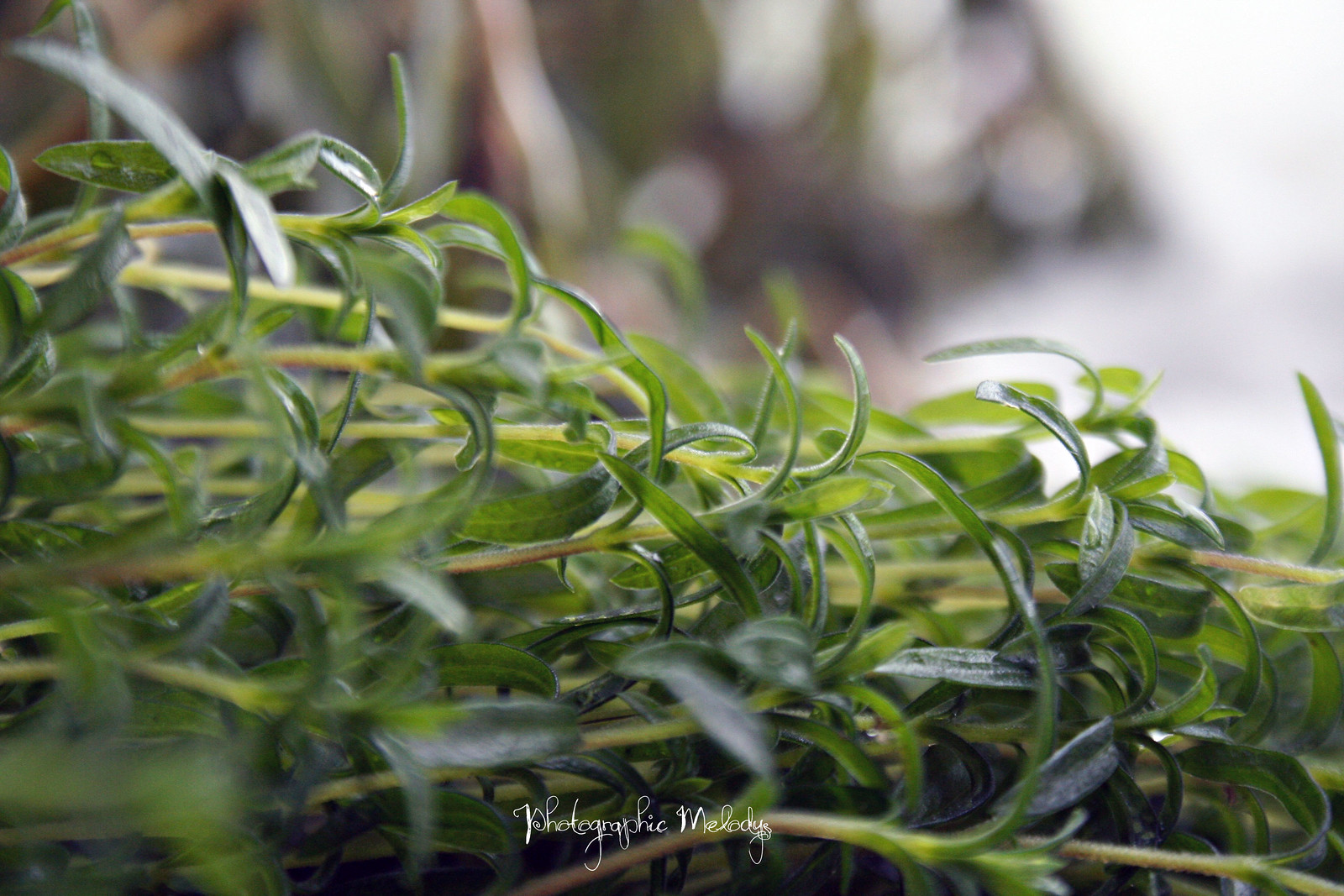This professional photograph showcases a close-up of an herb, likely rosemary or thyme, with thin, elongated green leaves. The composition captures the stems and leaves laying horizontally from left to right, with a focus on the middle ground of the herb plant while the foreground and background remain blurred. The colors in the image include various shades of green, yellow, white, and hints of black. The background features an indistinct, blurry object, emphasizing the greenery in the foreground. Positioned at the bottom center of the photograph is a small white text reading "photographic melodies." The setting appears to be an outdoor space, possibly a garden or park.